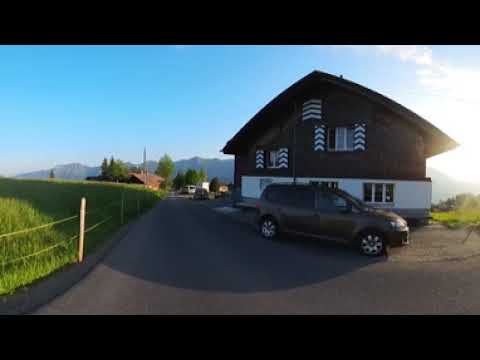A photograph captures a picturesque corner of a road, where a house stands prominently on the right. The house features a distinct two-tone exterior with the bottom floor painted white and the upper floor in brown. Enhancing its charm, the upper windows are adorned with chevron-patterned shutters in alternating white and brown, resembling upward-pointing arrows. In front of the house, a charcoal-colored van is parked, and sunlight from behind casts a warm glow over the scene. To the left, a basic fence comprising poles and strings encloses a grassy pasture. The road stretches straight ahead, revealing another house and a vehicle parked further along the right side. Further in the distance, a majestic mountain range rises under a clear blue sky, completing the tranquil rural setting.